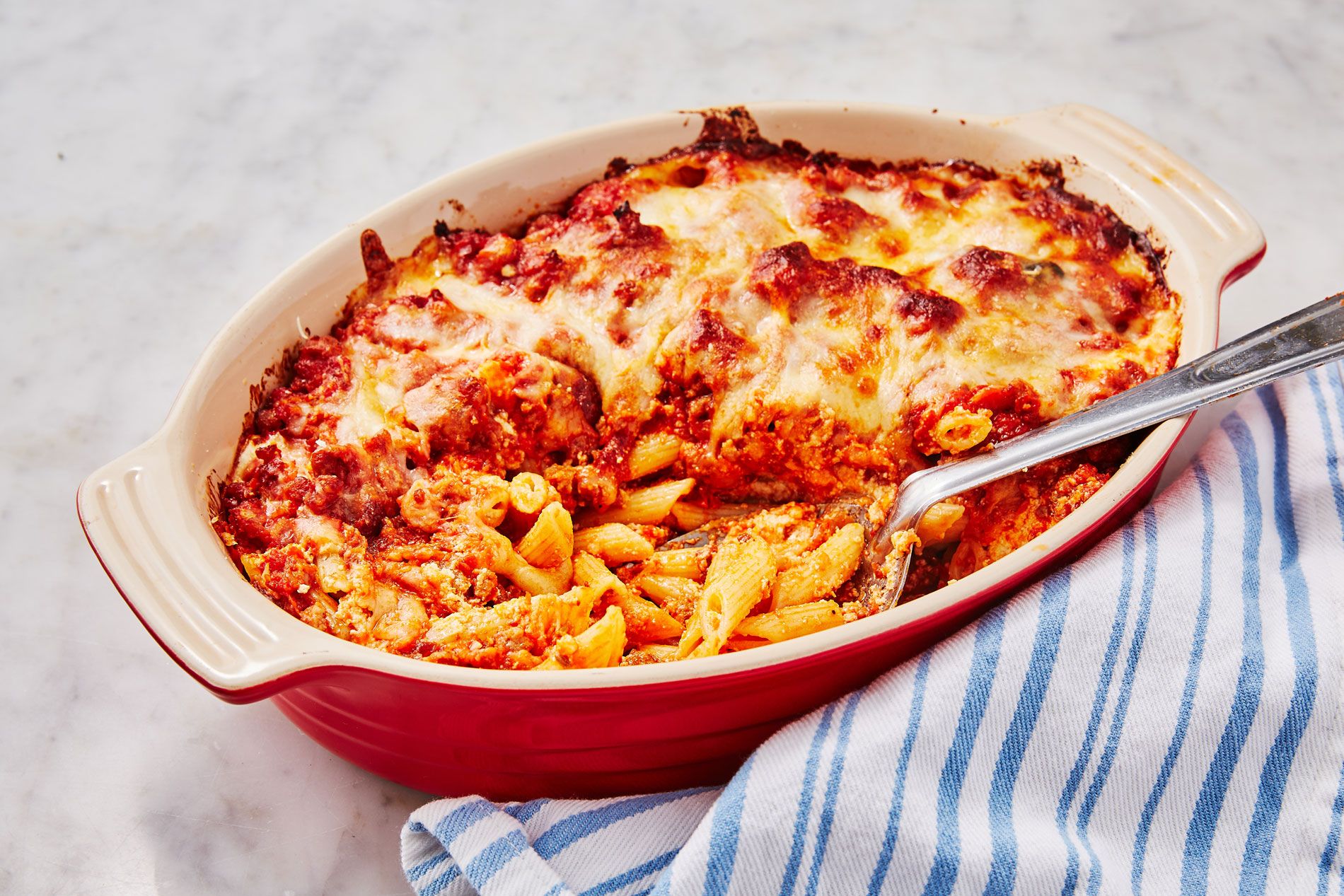The image features a delectable pasta dish, presented in an oval, oblong china crockery bowl. The bowl is striking with a red exterior and a beige or white interior and is equipped with two built-in handles. The dish sits atop a marble table, complemented by a blue and white striped tea towel positioned on the right side. The pasta within the bowl is a form of thick, ridged noodles, likely penne, generously covered in a rich tomato meat sauce. The surface is adorned with hard-baked cheese, slightly browned around the edges, alongside a layer of flakier cheese beneath. A large, distinctive spoon with an indented handle is plunged into the dish, poised as if ready for serving. It looks irresistibly delicious.